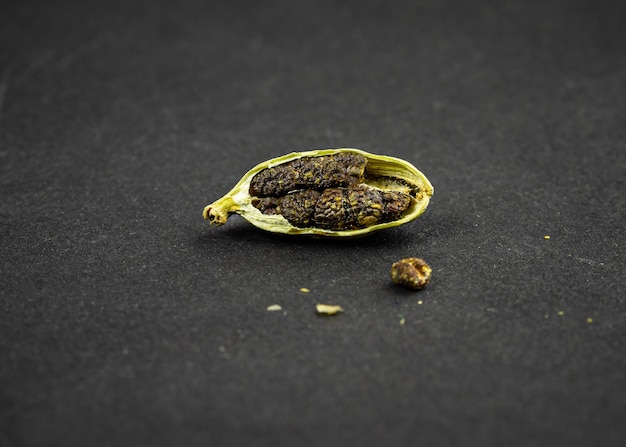This image depicts a close-up view of a seed pod that has been carefully split open and laid on its side. The pod, elongated and oval-shaped with a yellow-green exterior, reveals its interior filled with approximately seven dark, nearly black seeds that have a rough, brain-like texture. One seed appears to have fallen out of the pod, which is positioned on a dark black surface resembling velvet. Scattered around the seed pod are small pieces of plant material, likely remnants from when the pod was cut open. The inside of the pod exhibits a purplish or gray hue, contrasting against the vivid exterior. The detailed display highlights the intricate structure and texture of both the pod and its seeds.